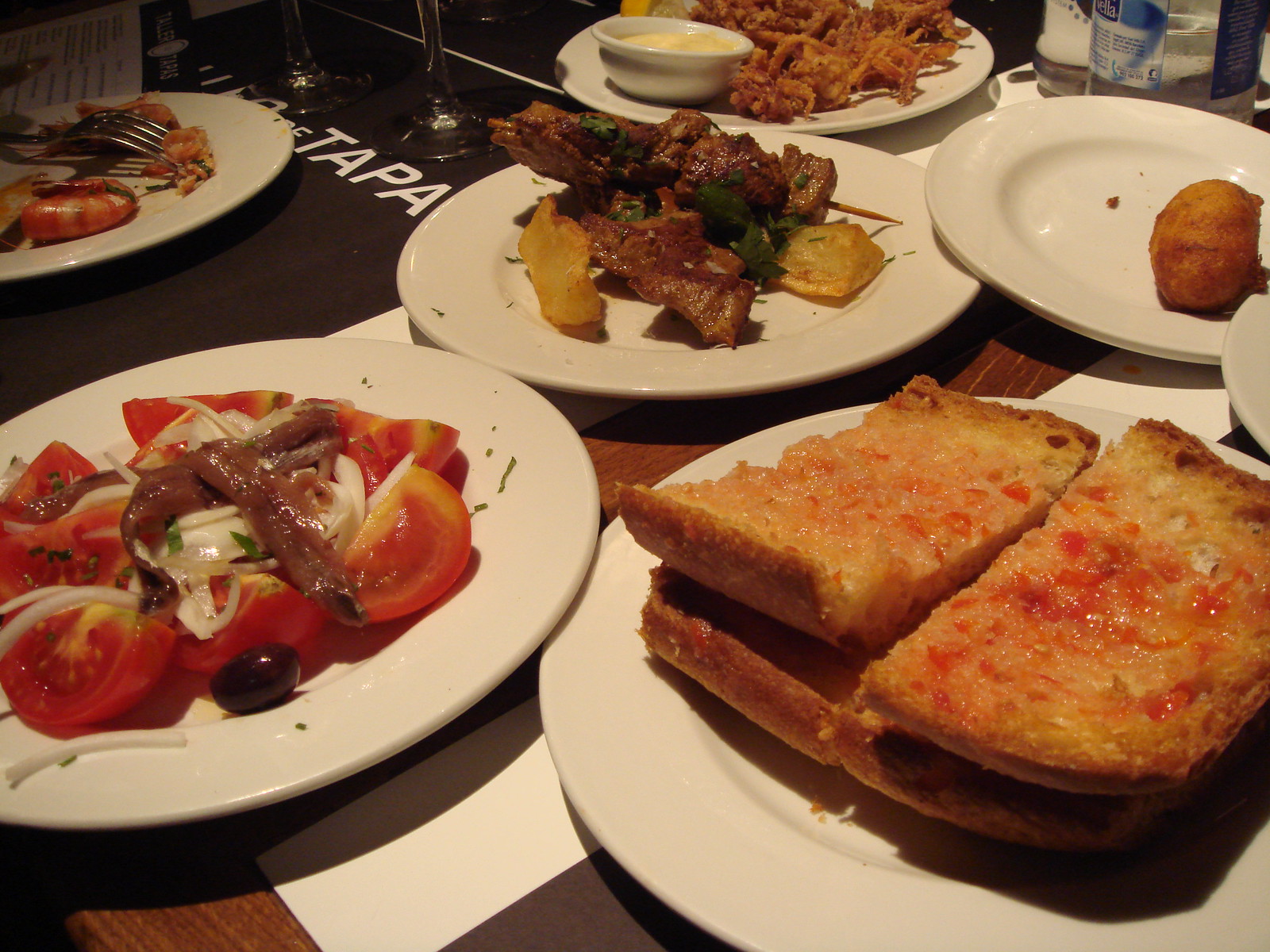The image depicts a spread of six distinct plates of food on a wooden table, presumably taken in a restaurant setting. Each plate is a white ceramic one, positioned casually across the table. There's a diverse array of foods featured:
- A plate of garlic bread topped with a red sauce or garnish, possibly accompanied by bacon.
- A plate with sliced tomatoes, onions, and olives, appearing to have some anchovies or meat.
- A plate with a skewer of meat garnished with parsley, and accompanied by either fried potatoes or lemon.
- Another plate holding shrimp, with some salad or garnish.
- A dish with noodles mixed with butter, labeled "Tapa".
- And in the back, a plate containing french fries and what looks like a fried roll or bun.

The scene includes a single placemat on the left side and a visible napkin, emphasizing the casual dining setup. The text "Tapa" suggests the plates are intended for sharing, typical of a tapas restaurant. The colors of the dishes range from vibrant reds and yellows to the more muted browns and greens, enhancing the visual appeal of the assortment.